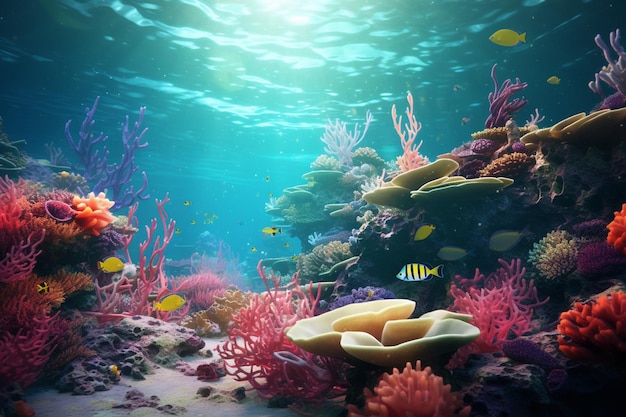This vibrant underwater scene, possibly an aquarium or ocean shot, presents a breathtaking view of the seabed teeming with diverse life. The turquoise blue water is illuminated by sunlight filtering down through its surface, casting a magical glow. Below, the sandy bottom is alive with a myriad of colorful marine flora and fauna. Splashes of orange, pink, purple, and red coral, along with off-white cone-shaped plants topped with dark-to-light green foliage, create a visually striking environment. Among the plant life, bright yellow fish marked with black fins and stripes swim gracefully, accompanied by additional yellow and blue-tinged fish. The water, shallow enough to see the rippling surface above, enhances the scene's vibrant, almost surreal quality, making it a vivid tapestry of underwater life.